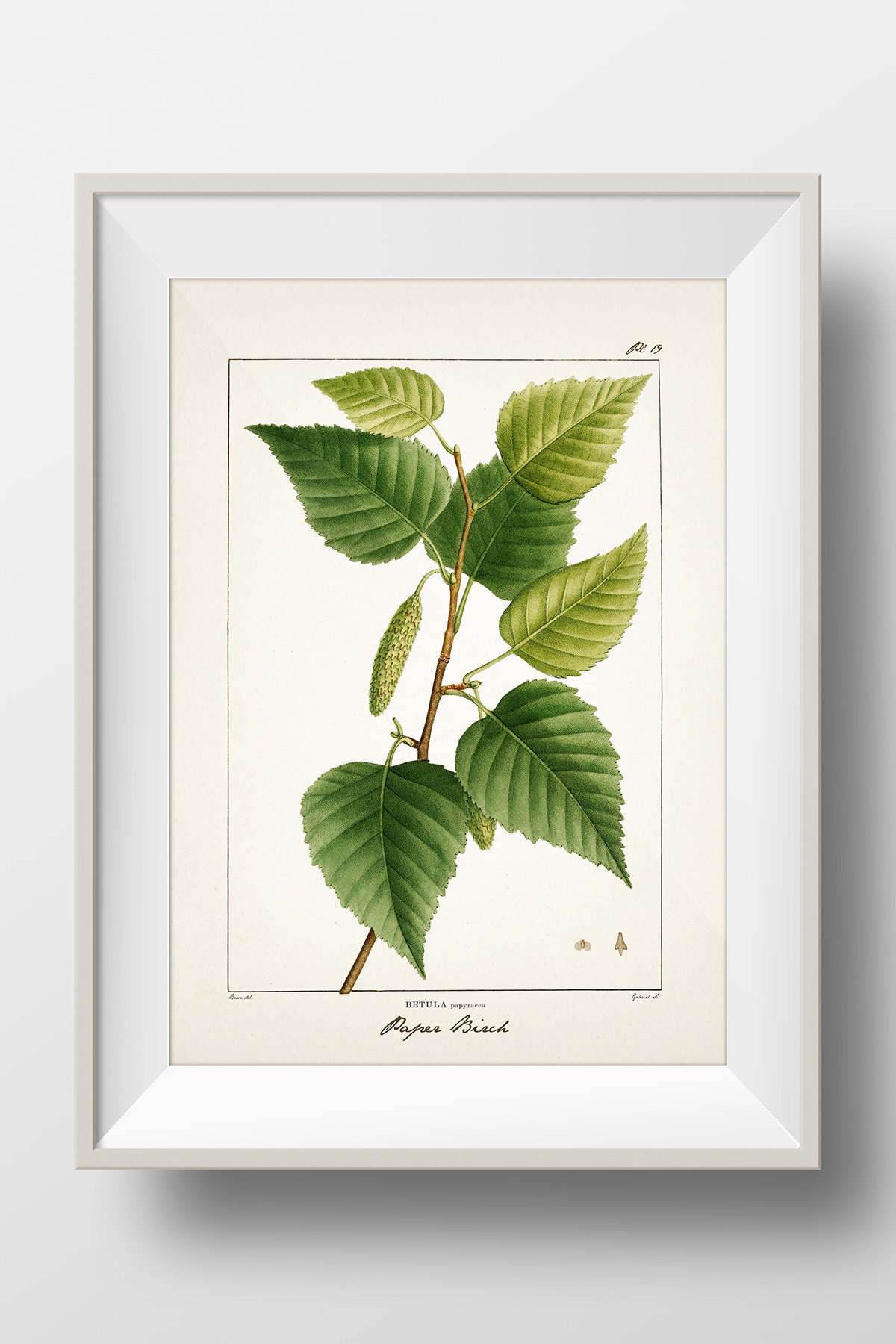This image features a photograph of a modern painting or illustration, set against a white background with multiple layered borders: an outer light grey border, an inner white border, a cream-colored border, and a thin black line closest to the artwork. The painting itself, encased in a white, rectangular frame that is vertically oriented, depicts a thin brown branch extending upward with seven green leaves of varying shades adorning it. Some leaves show hints of lime green, especially noticeable on the top three leaves. Additionally, a cocoon-like shape resembling a small piece of green corn hangs from the branch. Below the painting, although not clearly legible, there is some writing that appears to include the artist's signature.